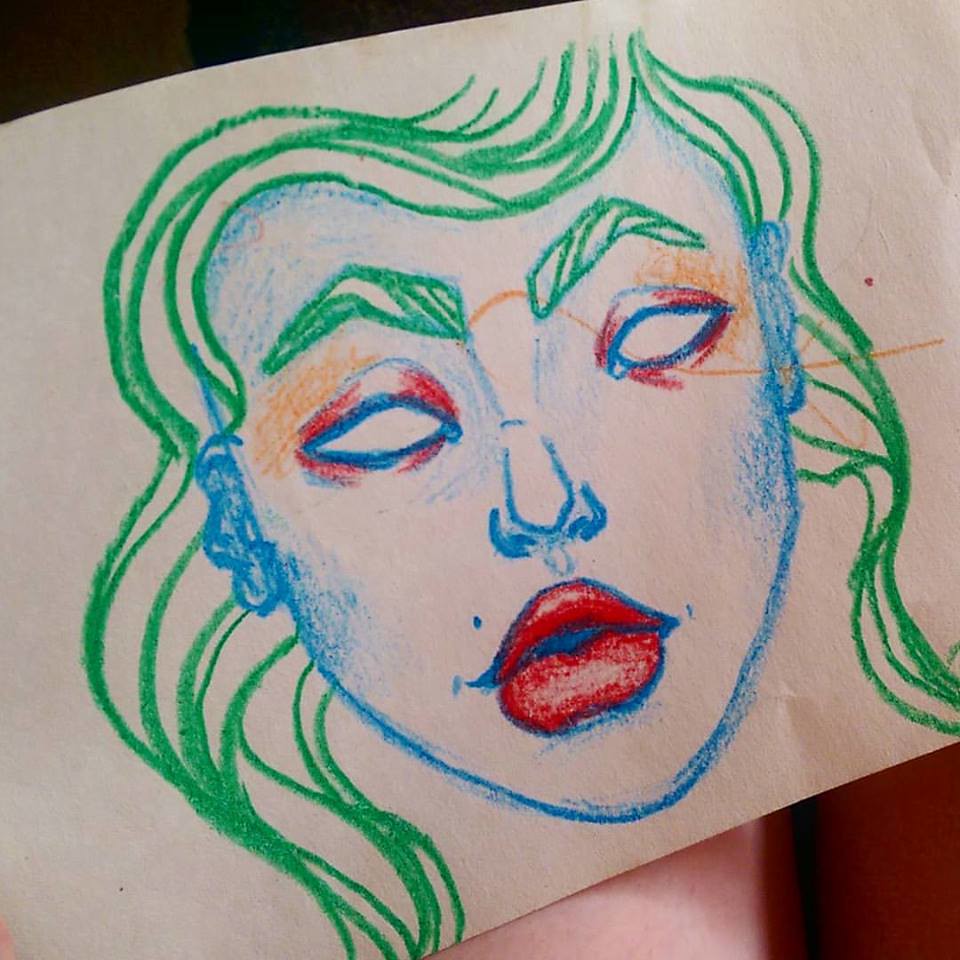This image captures a detailed sketch on a page, showcasing an intriguing and colorful face. The face, predominantly blue, features intricate blue outlines and subtle blue shading, giving it depth and character. Contrasting green, wavy hair frames the face, cascading down past the eyebrows, which are also green. The eyes stand out with blue outlines and a striking combination of red and orange shading, evoking a sense of vivid eye shadow. The nose is artistically rendered in blue, while the full, red lips add a bold touch to the composition. The drawing focuses solely on the face, omitting the neck and shoulders, ensuring all attention is drawn to the facial details. The background remains blurred, obscuring whether the sketch rests on a desk or someone's hand, thus directing the viewer's focus entirely on the colorful and captivating face.